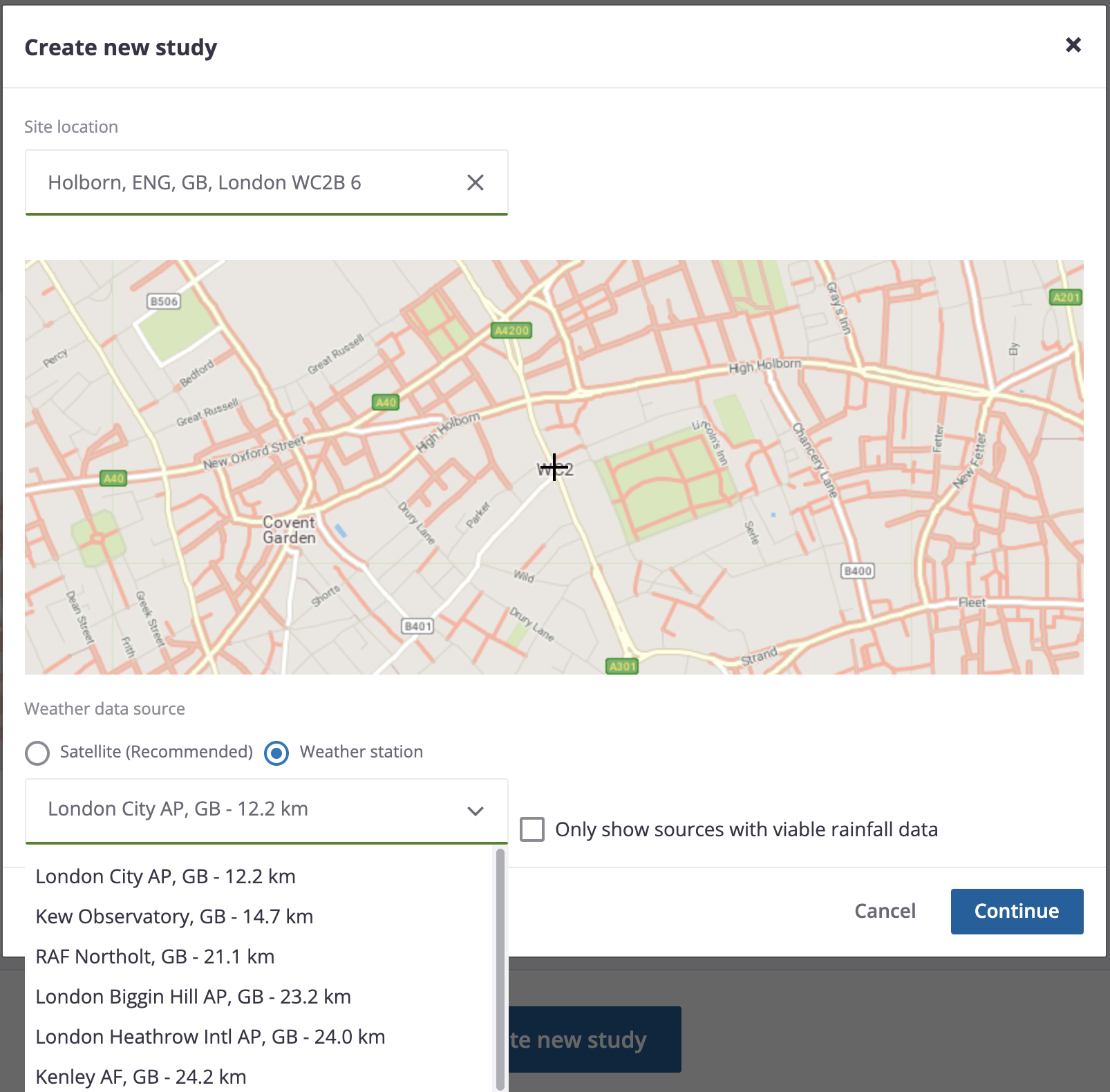The image depicts a webpage interface titled "Create New Study," with a specified site location of "Hulbourne, ENG, GB, London WC 2B 6." At the center of the interface is a map marked with a black cross, surrounded by prominent London streets, including New Oxford Street, High Hulbourne, and Clancy Lane. Covent Garden is labeled at the bottom left of the map. Below the map, there is a section labeled "Weather Data Source," offering two options: "Satellite" (recommended) and "Weather Station."

A dropdown menu is open, currently set to "London City AP GB 12.2 km," with alternative selections available such as "New Observatory GB 14.7 km," "RF Northolt GB 21.1 km," "London Biggin Hill AP GB 23.2 km," "London Heathrow International AP GB 24.0 km," and "Kenley AF GB 24.2 km." To the right of the dropdown is an empty checkbox option labeled "Only show sources with visible rain data." 

At the bottom of the pop-up are "Cancel" and "Continue" buttons. Behind this pop-up, there is a darkened area with a button labeled "New Study" at the end.